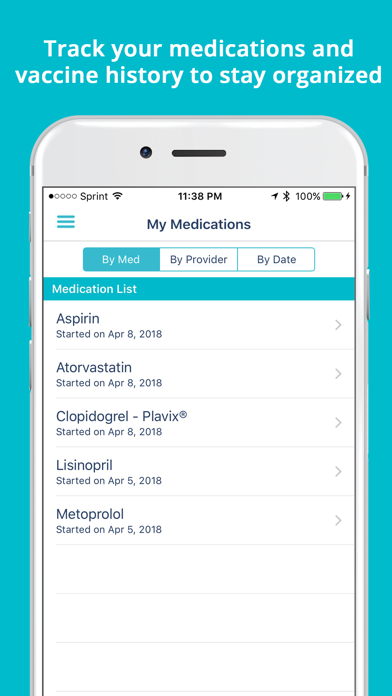This is an image of a smartphone screen displaying a medication and vaccine tracking app on a blue background. The status bar at the top of the screen shows the time as 11:38. The battery is fully charged at 100% and currently charging, indicated by a thunderbolt icon. The connection is displayed as Sprint with an active Bluetooth symbol.

The main interface features a header titled "Track your medications and vaccine history to stay organized." Below the header, there's an icon resembling a hamburger menu. The section is labeled "My Medications."

Within the app, several medications are listed with their respective start dates:
1. Aspirin - Began on April 8th, 2018.
2. Atorvastatin - Began on April 8th, 2018.
3. Cyprodryl, Plavix (CLOPIDOGREL) - Began on April 8th, 2018.
4. Lisinopril - Began on April 5th, 2018.
5. Metoprolol - Began on April 5th, 2018.

Each entry includes the name of the medication along with relevant details like start dates to help the user manage their medication regimen effectively.